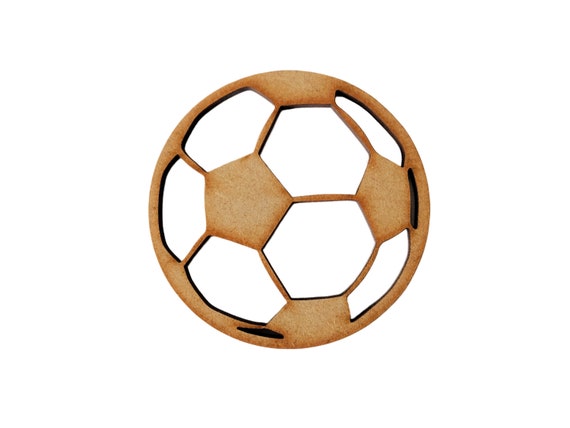The image depicts a flat, round piece of plywood, cleverly cut to resemble the design of a soccer ball. Set against a completely white background, the plywood features a series of hexagon and octagon shapes. There are four tan-colored wooden octagon pieces arranged centrally, connected by lines to seven surrounding hexagonal cut-outs that are either clear or transparent, allowing the white background to show through. The precision of the cut-outs gives the piece a 3D illusion, evoking the curvature typically seen on a soccer ball, despite being a flat, wooden object. Additionally, two small black spots are visible on the edge of the wood, adding minor, notable details to the overall minimalist design.